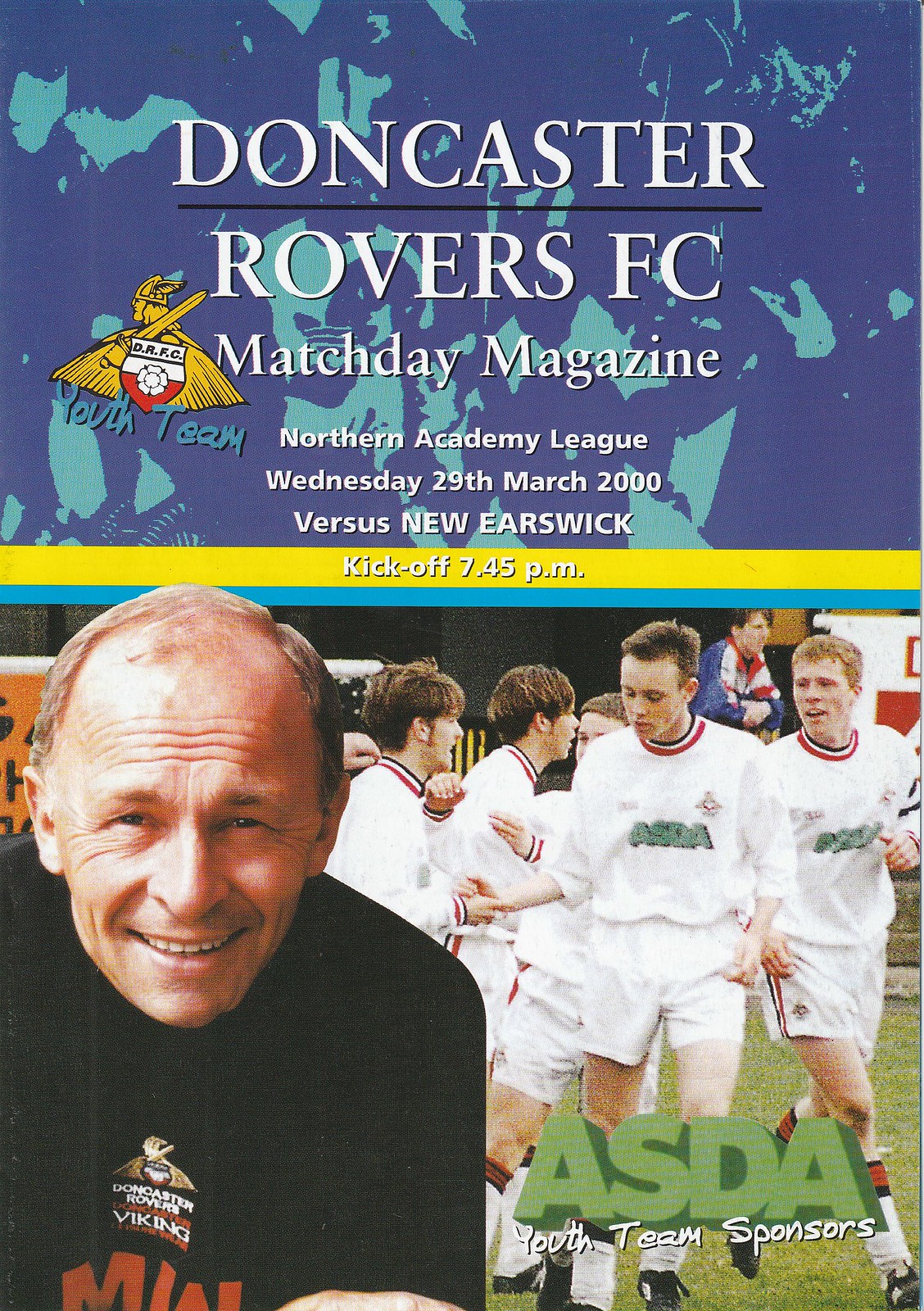This image is the cover of a Match Day Magazine for Doncaster Rovers FC. At the top, the title reads "Doncaster Rovers FC, Match Day Magazine." Below that, it indicates, "Northern Academy League, Wednesday, 29th of March, 2000, versus New Earswick, kickoff at 7.45 p.m." This text is placed on a blue background with a light blue, splotchy pattern.

The central portion of the cover features two linked photographs. On the left, there is an older man with a receding hairline and short hair, dressed in a black long-sleeve shirt, smiling with a wrinkled forehead. The shirt has the team name printed on the chest, suggesting he might be the coach. Behind him is an image of players in action, donning white uniforms with red and black collars and playing on a field. The text "ASDA Youth Team Sponsors" is printed underneath the photograph of the players.